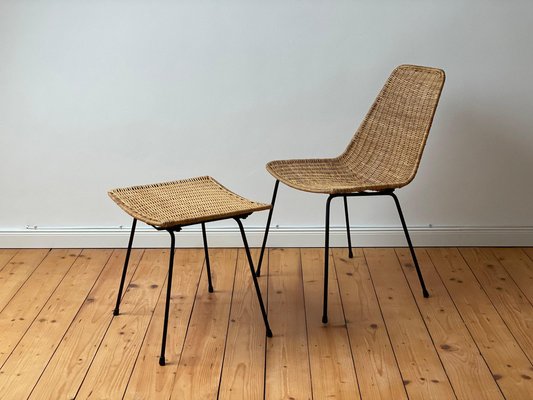This image captures a simple, yet refined furniture arrangement featuring a wicker chair and a matching ottoman. Both pieces are crafted with a traditional cane material where the body rests, giving a vintage feel reminiscent of 50s style furniture. The chair and ottoman have slender, black metal legs with rubber caps at their ends to prevent floor damage, adding to their minimalist, industrial aesthetic.

Centered in the image, the chair is oriented facing left and accompanied by the ottoman positioned perfectly for someone to rest their legs. They sit upon a warm, medium-brown wooden floor with darker knots adding character, and the background reveals a stark white wall, adorned only with some subtle electrical lines clipped along the skirting for a touch of understated detail. The overall composition is simple and uncluttered, with an elegant blend of traditional and modern elements.